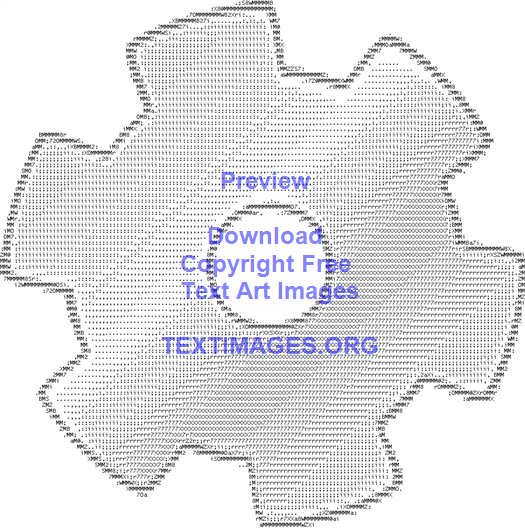The image displays a pixelated, black-and-white text art of a gear, resembling the output from an old matrix dot printer with its characteristic striped patterns in various shades of gray. The gear, which has six darker teeth, features a central white blank area encircled by a darker line. Overlaying the gear, in blue text, are the words: "preview, download, copyright-free text art images." Beneath this, on the fifth line, appears the textimages.org URL. This image, a sample from textimages.org, showcases their extensive collection of text art images available for free download, catering to art enthusiasts and students exploring digital art forms.